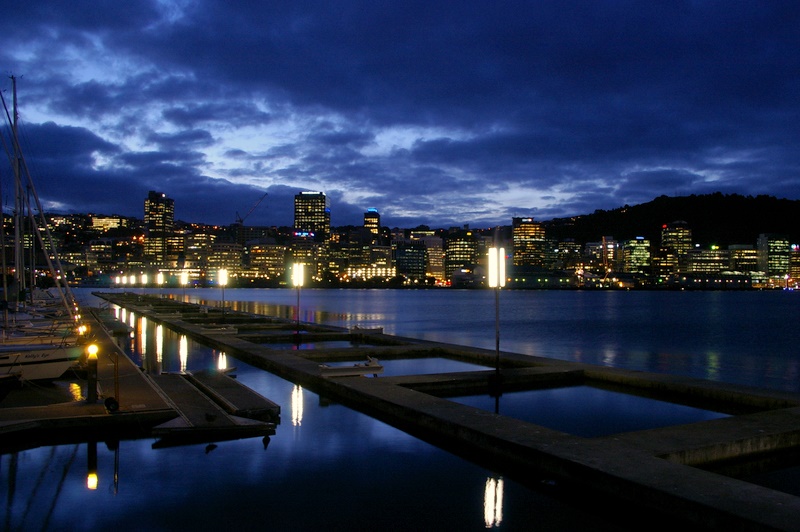This nighttime photograph captures a striking city skyline from the vantage point of a pier, featuring a dark, midnight blue sky partially obscured by light white clouds. The cityscape includes several large illuminated buildings, suggesting a medium to large-sized city. Notably, the top right-hand corner of the image reveals a hill. The foreground presents a marina on the left, with multiple rows of boats, primarily sailboats, docked in their slips. Toward the center of the photo, there are cement squares extending into the water, resembling a pier. The river, reflecting a deep blue hue, gracefully cuts through the scene, while a lit-up bridge adorned with lights adds a touch of brilliance, beautifully contrasting with the dark sky and city lights.